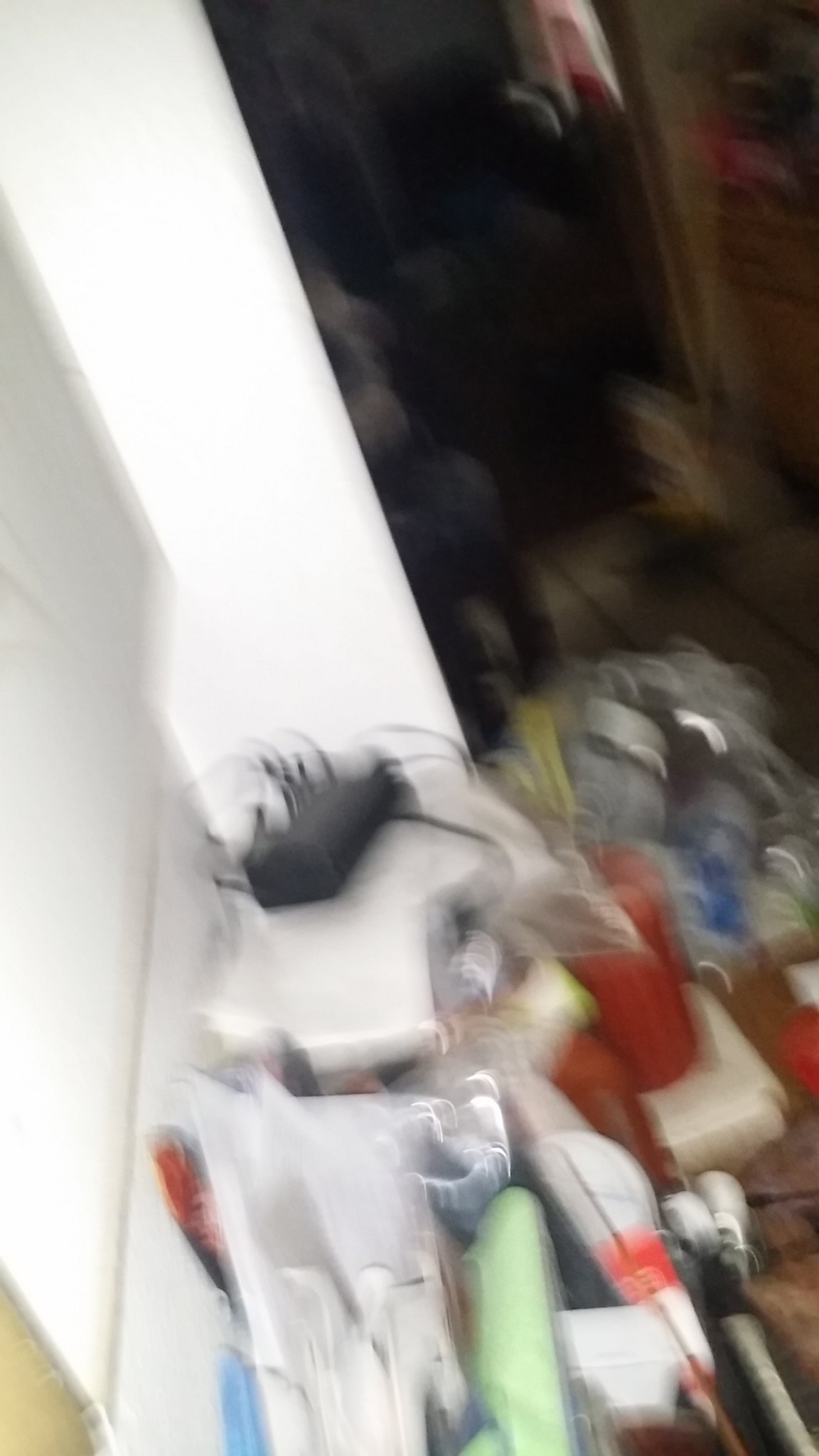This image is a blurry photograph that appears to be taken inside someone's home. On the left side, there is a discernible white wall. In the upper right corner, there's a dark area with indistinguishable blurred objects. The foreground is cluttered with various items, making it difficult to identify specific objects. There is a visible pile of items where colors can be faintly distinguished. On the right-hand side, there seems to be a bag containing silver objects. To the left of this bag, a white object with a black rectangle and wires is noticeable. Further to the right, a red cup or container stands out. Additionally, in the forefront, there appears to be a white piece of paper or possibly a bag.